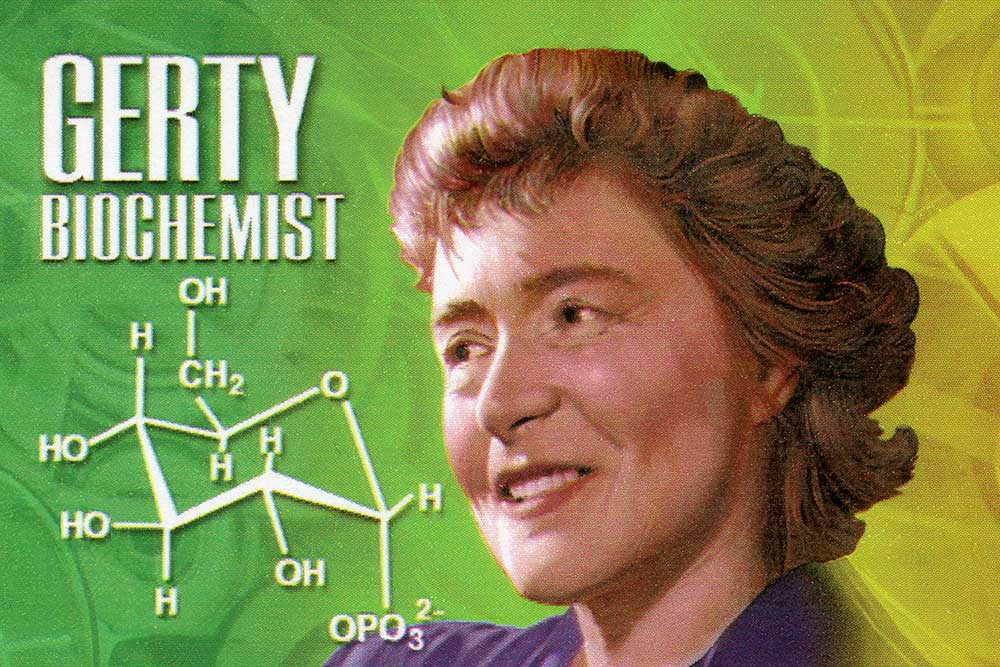The image appears to be a detailed, colorized drawing from what might be the 1940s or 1950s. It features a woman named Gertie, identified as a biochemist, indicated by the text “Gertie, biochemist” at the top left. Gertie has reddish-brown, short hair styled in an old-fashioned manner and is wearing a purple shirt. She is shown with a slight smirk or half-smile, looking towards the left side of the image. The background is a design resembling chemical or mechanical elements in green and yellow hues. In the lower-left portion of the background, there is a model of a chemical composition, showing connected elements, with labels like O H for oxygen and hydrogen atoms.